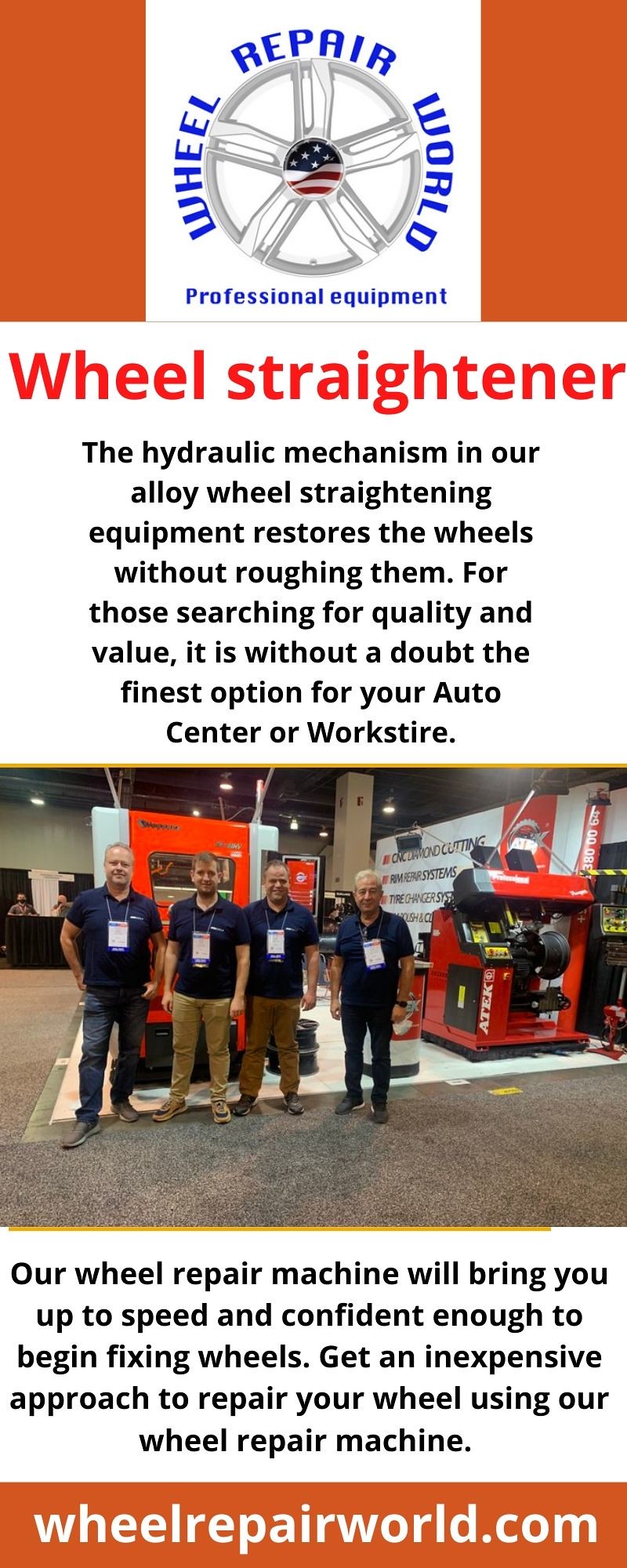This vertically aligned rectangular poster from Wheel Repair World prominently features their circular logo with blue all-caps text and an image of a silver car steering wheel with an American flag design. The top section, bordered in orange with a white center, includes the logo and the words "Professional Equipment." Beneath, in red letters against a white background, "Wheel Straightener" is boldly displayed, followed by detailed black text explaining, "The hydraulic mechanism in our alloy wheel straightening equipment restores the wheels without roughing them. For those searching for quality and value, it is without doubt the finest option for your auto center or work star." The image also showcases four men in a mechanic shop, each wearing navy blue polos and either jeans or brown pants, along with lanyards. They stand amidst mostly red machinery on a concrete floor. More black text below highlights the benefits of their wheel repair machine, concluding with, "Our wheel repair machine will bring you up to speed and confident enough to begin fixing wheels. Get an inexpensive approach to repair your wheel using our wheel repair machine." At the very bottom, an orange rectangle with white lettering displays the URL "WheelRepairWorld.com."